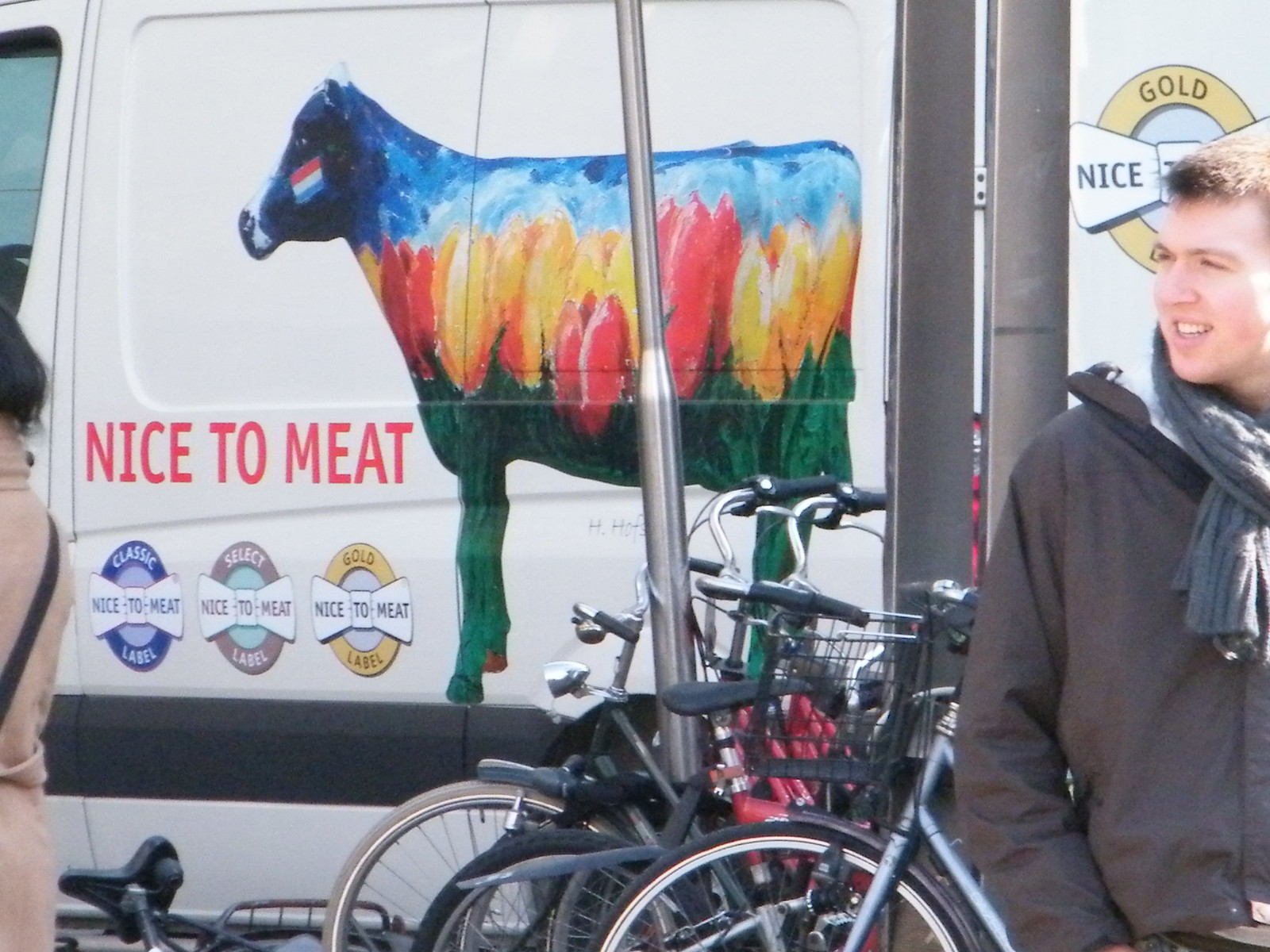The photograph captures a dynamic outdoor scene centered around a distinctive white van parked by the side of a road. The van features a unique, photorealistic tie-dye cow adorned with vibrant yellow and red tulips painted on its side. Prominently displayed on the van are the words "Nice to MEAT" in red letters, along with three gold circular logos below that read "Nice to MEAT Classic Label." 

In the immediate foreground, a collection of three bicycles is lined up next to a pole, adding to the lively atmosphere. To the right of the image stands a white man, wearing a dark gray winter coat and a gray scarf, looking towards the left with a slight smile, revealing his upper front teeth. He has short dark hair and a light skin complexion. On the far left, the backside of a person is partially visible; this individual, seemingly a woman with dark hair, is wearing a long tan (or peach-colored) coat and carrying a black-strapped bag over their shoulder, walking off-frame.

The setting is bathed in daylight, indicating that the photo was taken on a bright, clear day, emphasizing the colorful details on the van and the cheerful mood of the scene.